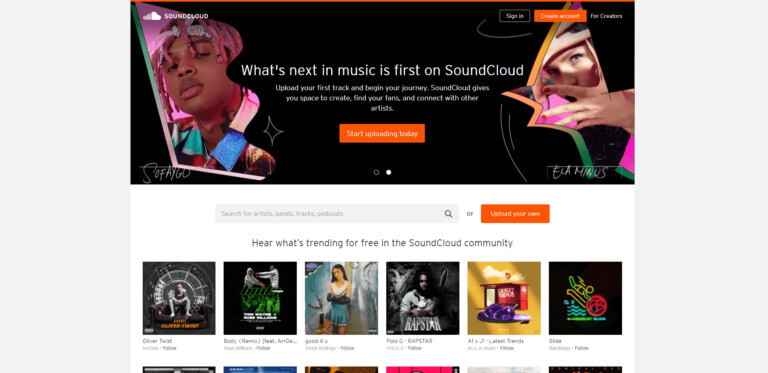This is a screenshot of the SoundCloud website. The top left corner prominently features the SoundCloud logo, accompanied by an icon of a cloud. On the top right are options for "Sign In" and "Create Account for Creators."

A prominent black banner spans across the page, showcasing two photographs. The left photograph depicts a dark-skinned person with blonde twists and a Mickey Mouse tattoo on their neck. They are dressed in a vibrant, multicolored collared shirt with the name "Sofaygo" (S-O-F-A-Y-G-O) displayed underneath. The right photograph features a woman framing her eyes with her fingers, with the name "Elaminus" (E-L-A-M-I-N-U-S) below her.

The banner bears the tagline: "What's next in music is first on SoundCloud. Upload your first track and begin your journey. SoundCloud gives you space to create, find your fans, and connect with other artists. Start uploading today."

Below the banner, there is a search bar with the prompt: "Search for artists, bands, tracks, podcasts, or upload your own." 

Highlighted tracks under "Hear what's trending for free in the SoundCloud community" include:
- "Oliver Twist" (followed by an unreadable text)
- "Body Remix"
- "Good For You" by Olivia Rodrigo
- "Rap Star" by Polo G
- Another track that is too blurry to discern

The section titled "Latest Trends" ends with the title "Slide."